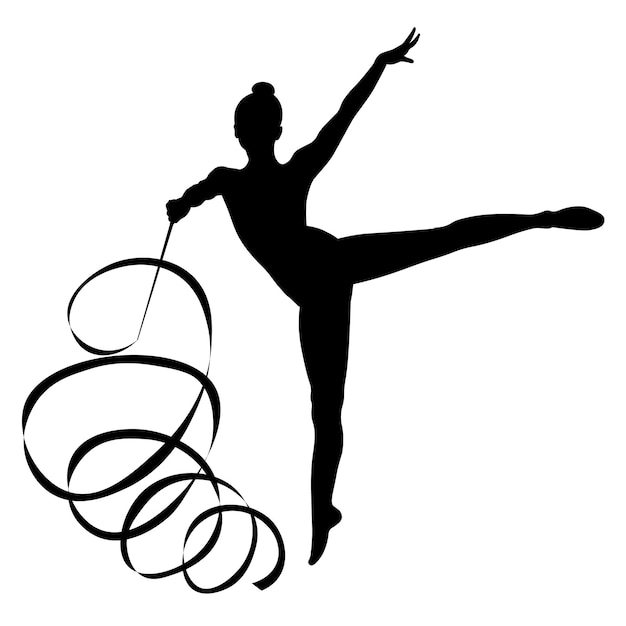In this striking black silhouette on a white background, we see a graceful ballerina or gymnast. She stands elegantly balanced on the toes of her left foot while her right leg extends straight back behind her at a dramatic angle. Her right arm reaches upward and outward at a 45-degree angle, with her palm facing upward, while her left arm holds a long, looping ribbon used in rhythmic gymnastics. The ribbon forms a series of five or six loops, spiraling down near her standing foot. Her hair is styled in a bun, and her face is turned completely away from the viewer, adding a sense of mystery. The simplicity of the monochromatic design emphasizes her poised form and the flowing motion of the ribbon, suggesting it could be part of a logo or advertising campaign.